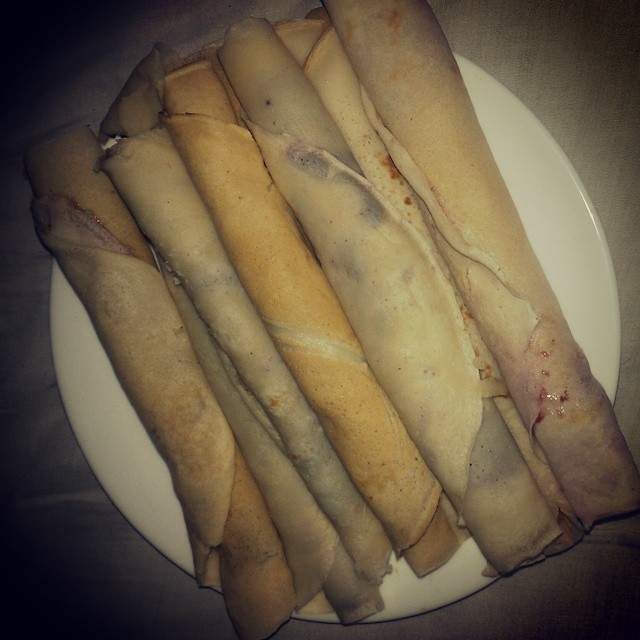The indoor color photograph is a close-up shot taken from above, capturing a round, white ceramic plate placed on a white table. On the plate are five rolled food items that resemble tortillas or crepes, varying in color from light tan to darker yellow. Each item is meticulously prepared and remains untouched. The rolled items, which span the length of the plate, appear to be wrapped in a tortilla-like or pancake shell. One end of a roll has a white substance sticking out, possibly sour cream, while another seems to contain a jelly or sauce. The dish's details, captured in the darker lighting of the foreground and sides, suggest a savory and potentially sweet filling, hinting at a breakfast crepe dish.